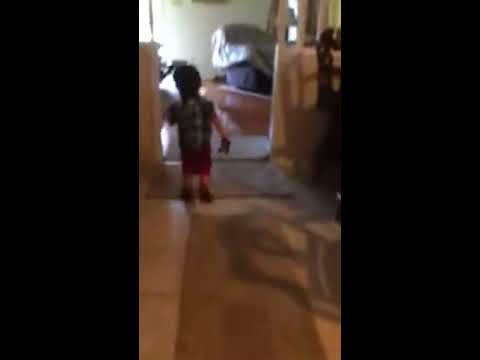The image is a small, square photo framed by thick, black vertical borders on both sides, each taking up around a quarter of the image. The central portion, though quite blurry, depicts a toddler—likely around two or three years old—walking away from the camera and towards a different room. His outfit includes red shorts and possibly brown shoes. He appears to be holding something in his right hand, and has dark hair, which may be black or brown. There’s an ambiguity about whether he has a backpack or not. 

At the bottom of the image, there’s a light brown rug, seemingly on top of an off-white tile floor. The child is approaching a doorway that leads into a room with a white wall. Within this room, various items are visible; there may be a blue chair near the living area and a tan carpet runway leading further inside. The left side of the room shows a kitchen chair pushed against a table, while the right side features various objects piled up, with some curtains visible in the top right corner. A ledge or countertop with white wood molding is discernible to the child’s left as he moves towards the room. Overall, the lack of clarity in the image makes further detailed recognition difficult.